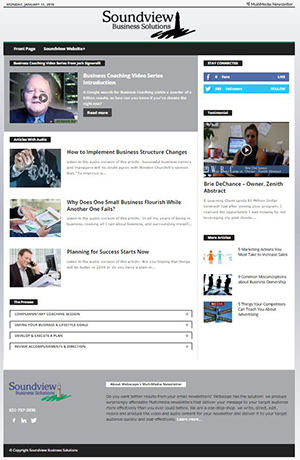This image is a detailed screenshot of a webpage. The page features a mid-grey bezel. Centrally, the text reads "Sound View," with "Business Solutions" positioned just below it. There is a prominent lighthouse grahic with a black squiggle beneath it.

On the extreme right and left sides of the page, there is small, unreadable black text. The image contains several distinct sections. 

The top portion displays an elderly man with short white hair sitting atop what appears to be a television or monitor.

Below this, there is an illustration of a person drawing on a clear whiteboard using a white marker. The text adjacent to this segment reads, "Why does one small business flourish while another one fails?" Additional text following this indicates, "How to implement business structure changes."

At the bottom section of the page, the text states, "Planning for success starts now," accompanied by an image of a man in a sharp black tuxedo and white dress shirt, his attire giving an illusion of being black in the screenshot. He holds a black phone in his right hand and has short brown hair.

In the page's footer, on the very bottom left-hand side in dark blue text, "Sound View" is visible. Near this text is a detailed graphic of a lighthouse, colored brown and blue, standing on a patch of grass.